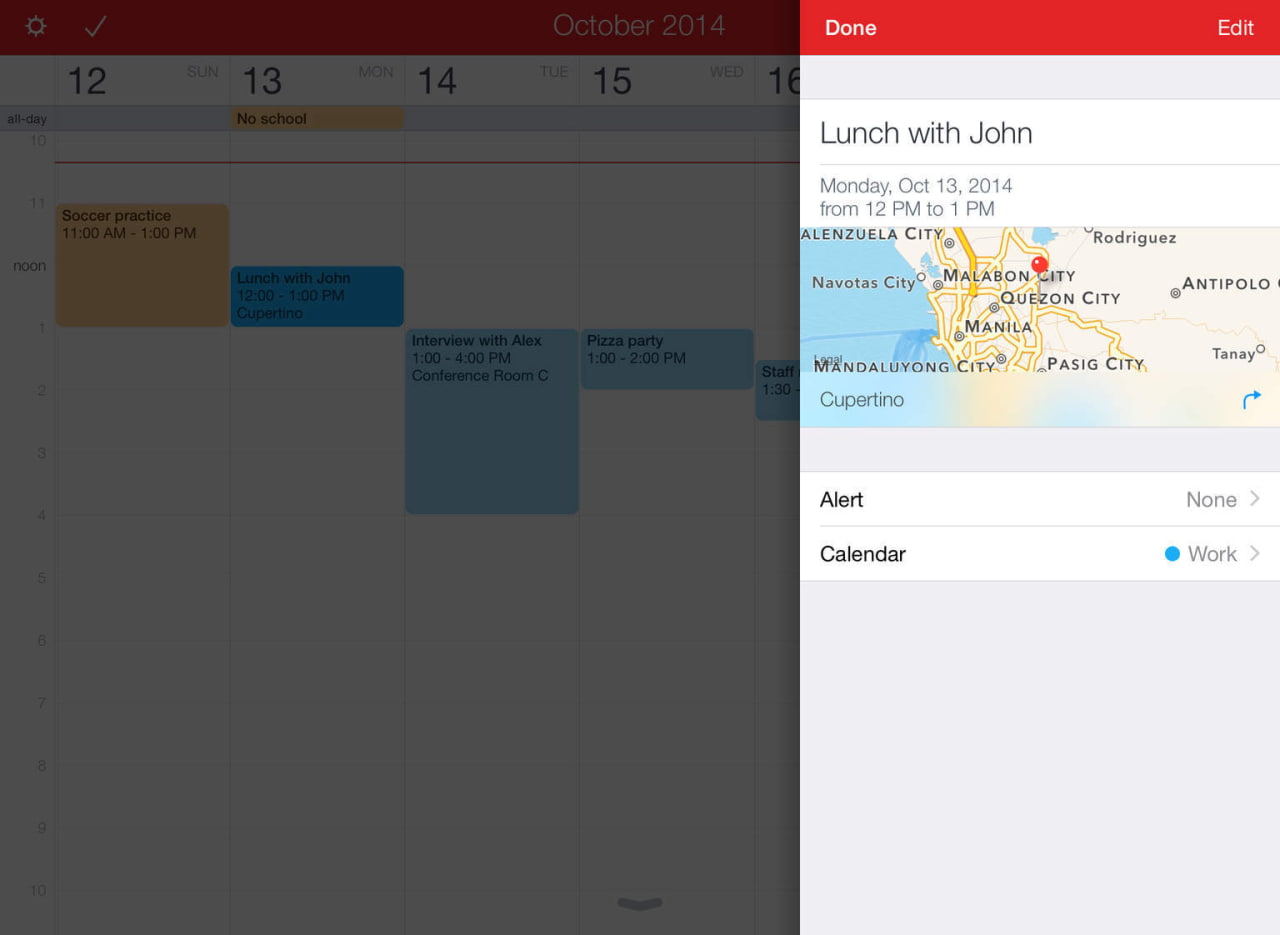The image showcases a digital calendar interface on the left, slightly darkened, displaying dates and planned events. The top of the calendar panel reads "October 2014," with visible dates from 12 to 16 prominently displayed. Notable entries include "Soccer Practice," "Lunch with John," "Interview with Alex," and "Pizza Party."

On the right, there's a detailed reminder section highlighted in red. At the top of this section, options "Done" and "Edit" are visible, suggesting the user can mark the task as completed or make changes. Below, the reminder details a scheduled event, "Lunch with John," set for Monday, October 13th, 2014, from 12 PM to 1 PM. Accompanying this reminder is a map marked with various labels such as Manila, Quezon City, Malabon City, Nevada City, Rodriguez, Antipolo, Mandaluyong City, Pasig City, and Tanay. The map features yellow lines indicating streets or routes and a small red thumbnail pinpointing a specific location. Additionally, water bodies are seen on the left side of the map.

The reminder section further shows an alert setting labeled as "None" and a categorical marker, "Calendar," indicating the activity is linked to the "Work" calendar, represented by a blue dot.